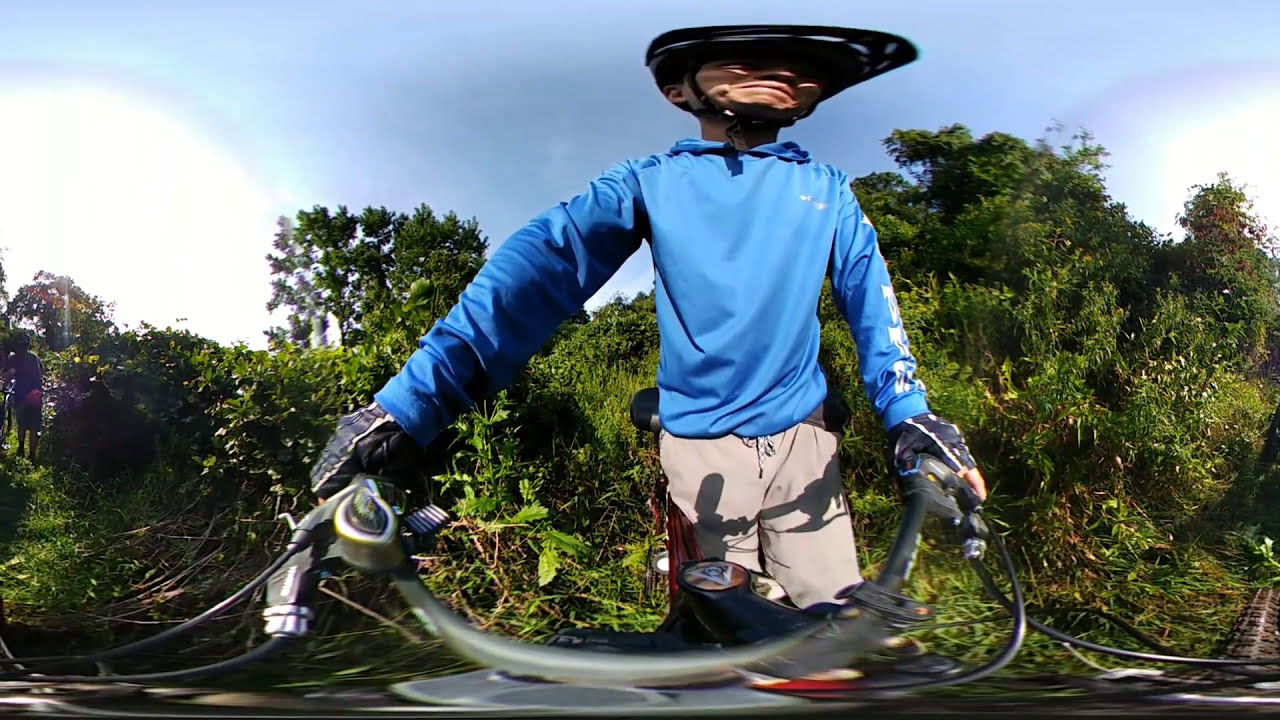The image captures an older man, possibly of Asian descent, riding a motorized bike or mountain bike through a lush, grassy undergrowth on a bright, sunny day with no clouds in the sky. He is wearing a helmet and a blue long-sleeved hoodie adorned with white designs on the left arm. His khaki drawstring pants or shorts complement his black gloves. The handlebars, also black, are positioned at handlebar level, with the camera angle panning up to his face. The man, who has a relatively normal build, appears to look upwards rather than at the camera. Behind him, there is an abundance of grass, bushes, and trees. The 360-degree panoramic image shows a slightly distorted view at the bottom, with the front tire of the bike visible, seemingly moving along a flattened path in the underbrush.